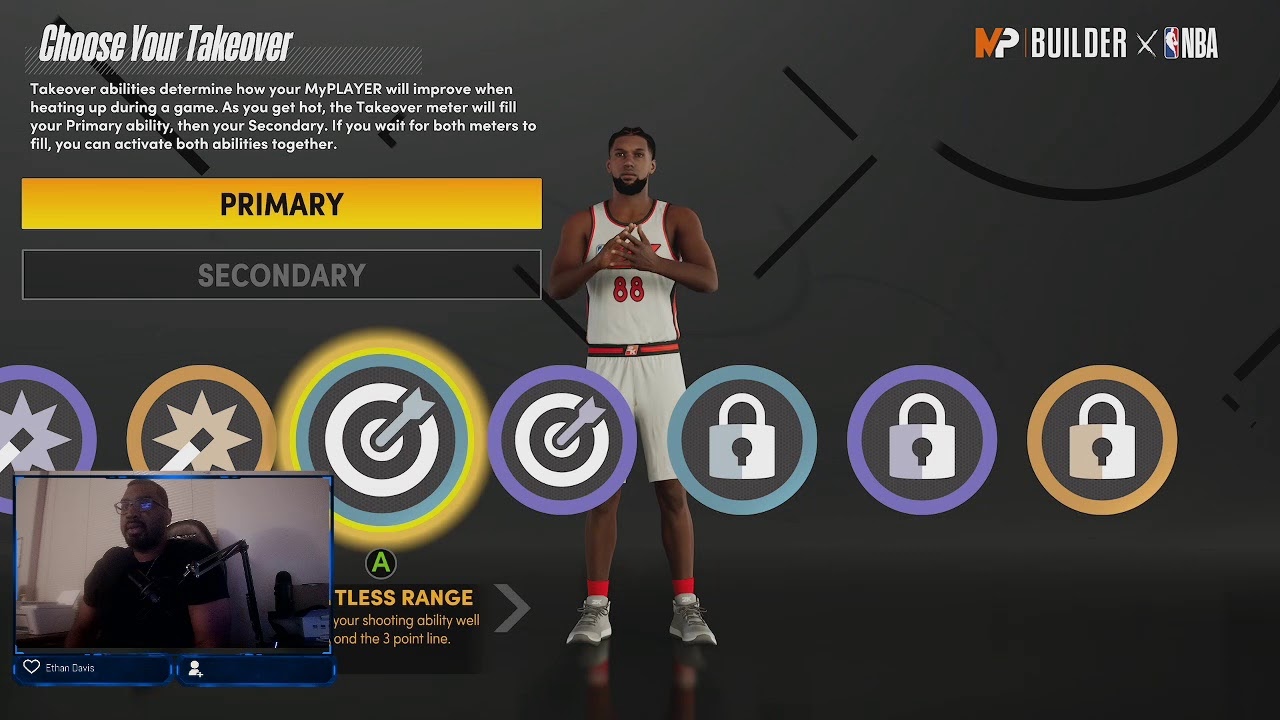In the image, we see a detailed interface from a sports game setup, likely related to NBA. The background is a black field, which prominently displays text on the left-hand side. The white text reads: "Choose your takeover. Takeover abilities determine how your MyPlayer will improve when heating up during a game. As you get hot, the takeover meter will fill your primary ability, then your secondary. If you wait for both meters to fill, you can activate both abilities together." Below this text, there's a line along with a button labeled "Primary," which is colored yellow with black font. Adjacent to it is another button labeled "Secondary," displayed in black with green font.

On the right side of the screen, there's a character model of a player. The player is an African American man wearing a white tank top with red lettering displaying the number "88." He also has white shorts, gray and white tennis shoes, and white and red socks. The character has short black hair and a neatly trimmed short beard beneath his chin.

Above the player, the text "MP Builder x NBA" is displayed. Surrounding the edge of the interface are colorful circles in various hues of purple, orange, yellow, and green. These circles contain different icons: stars, bullseyes, and locks, with a distribution of two stars, two bullseyes, and three locks.